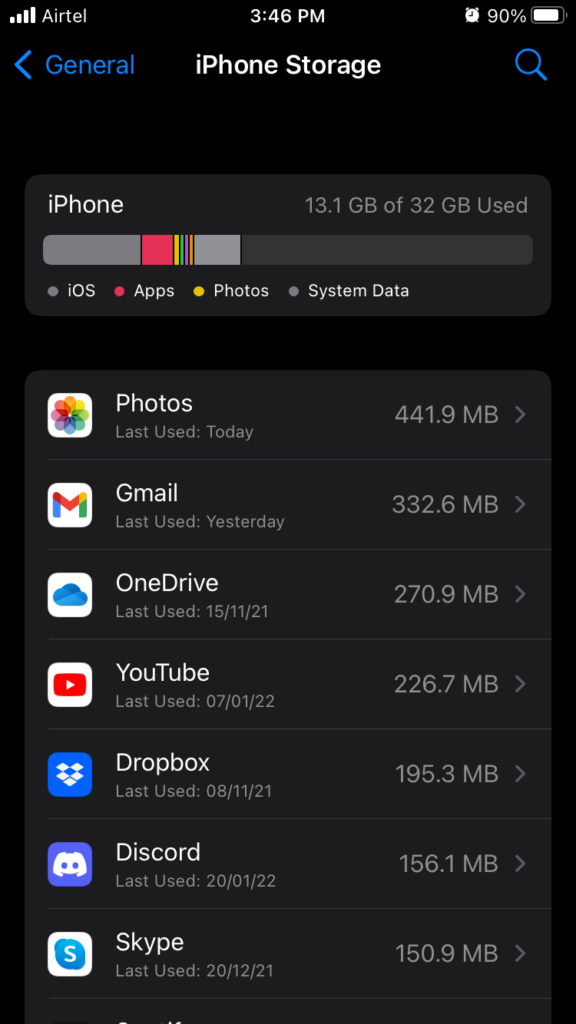This detailed screenshot from a cell phone displays various elements prominently:

- **Top Left Corner:** The coverage icon signifies a connection with the provider "Airtel." 
- **Time and Status Bar:** The time is marked at 3:46 PM, with the battery at 90% and an active alarm set.
- **Navigation Bar:** A blue arrow pointing left accompanies the word "General" in blue letters.
- **Section Title:** "iPhone Storage" is displayed in white text.
- **Search Icon:** A magnifying glass icon for search functionality is located on the right side.
- **Storage Information:** The phone shows 13.1 GB used out of the available 32 GB of storage. 
- **Categories Listed:** iOS, apps, photos, and system data are mentioned as categories.
- **App Usage Details:**
  - **Photos:** Last used today, using 441.9 MB.
  - **Gmail:** Last used yesterday, with a space usage of 332.6 MB.
  - **OneDrive:** Last accessed on 15/11/21, using 270.9 MB.
  - **YouTube:** Last used on 7/1/22, consuming 226.7 MB.
  - **Dropbox:** Last accessed on 8/11/21, using 195.3 MB.
  - **Discord:** Last used on 20/1/22, with 156.1 MB used.
  - **Skype:** Last accessed on 20/12/21, utilizing 150.9 MB.

The image itself is taller than it is wide and does not contain any people in the captured screenshot.